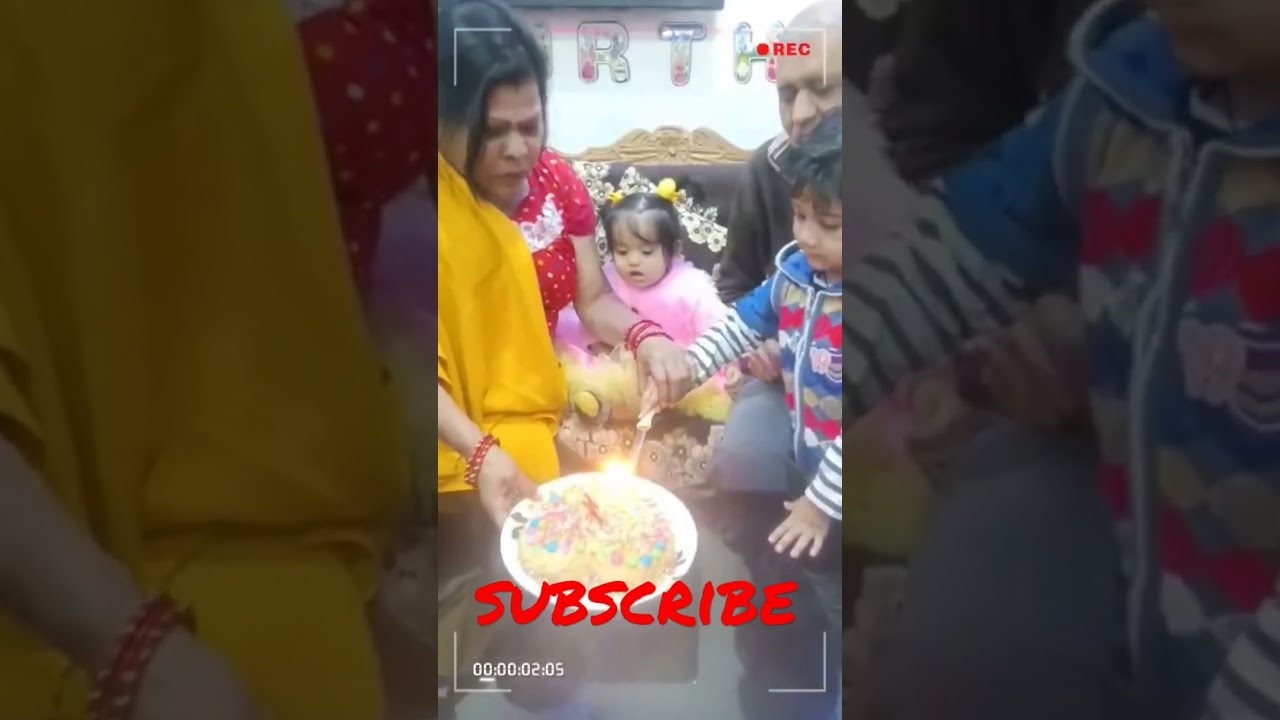In this vivid outdoor scene, a family is captured in the midst of a joyful birthday celebration under the midday sun. Centrally positioned in the image is a white, circular bowl containing a vanilla cake adorned with multicolored sprinkles, which the young boy is intently lighting. The boy, dressed in a blue, white, red, and yellow sweatshirt, stands close to the cake with assistance from an older, bald man wearing a black shirt with a white collar. 

To the left, a woman with dark black hair pulled back, wearing a red and white polka-dotted dress and a mustard throw over her shoulder, observes the scene proudly. Red bracelets adorn both of her wrists, adding to her vibrant appearance. Sitting near her is a toddler, approximately two years old, dressed in a fluffy pink sweater with her hair styled in two pigtails.

Above the family, the backdrop reveals the exterior of a building, suggesting that this heartfelt celebration is taking place in their backyard. The word "subscribe" is prominently displayed in red at the bottom center of the image, accompanied by a timer reading "2:05". Additionally, the top right corner includes a red recording symbol, indicating the moment is being documented, perhaps for posterity or social media.

This photograph beautifully encapsulates the warmth and togetherness of a family's special day, meticulously framed with each member playing a significant role in the celebration.